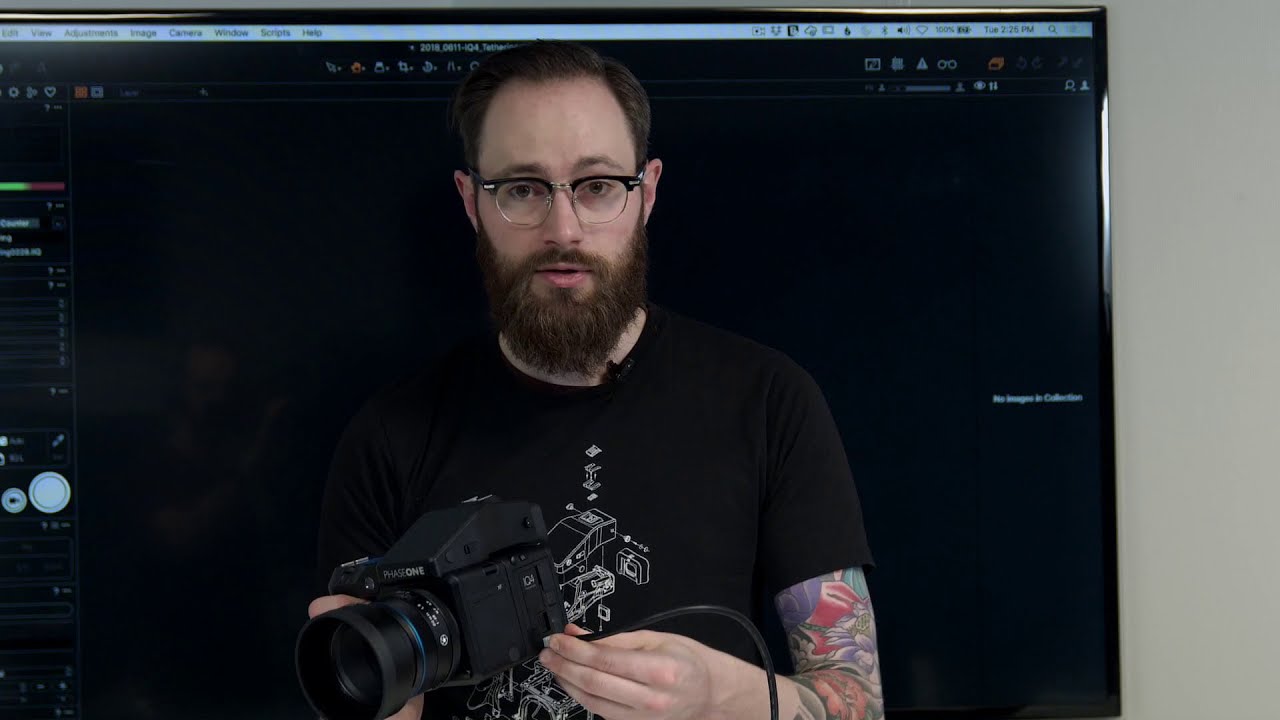The image is a detailed still shot, possibly from a video, prominently featuring a middle-aged Caucasian male with dark hair, a receding hairline, and a beard and mustache. He is standing in the center, directly facing the camera and wearing black-rimmed glasses. His attire includes a black t-shirt adorned with a technical white graphic, depicting a disassembled camera, which adds an ironic touch considering the camera equipment he is handling. His left arm, which sports an extensive tattoo from the sleeve to the wrist, is bent at the elbow, pointing towards a black camera labeled "Phase One" with an elongated lens that he holds in his right hand. It appears he is about to plug a black cord into the camera, suggesting he could be demonstrating or instructing on its use. The background is predominantly black with traces of what looks like imaging software, perhaps Photoshop, open on the computer screen. On the far left edge of the image, there are horizontal color bars and a light blue circle subtly present against the black backdrop.